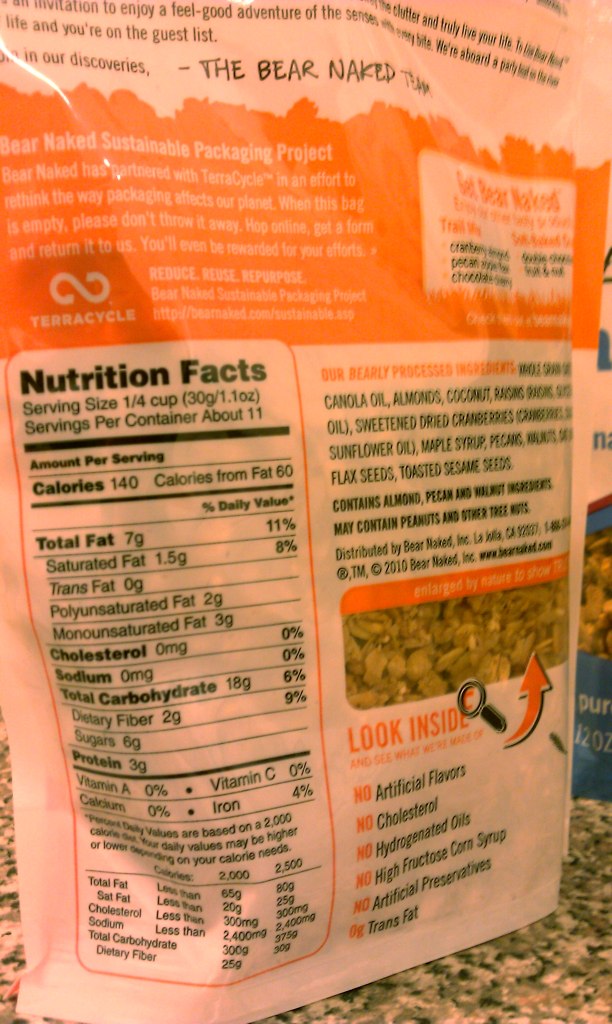The image depicts the back of a package of Bare Naked granola. The top of the package features an orange and white section dedicated to the Bare Naked Sustainable Packaging Project, providing details about the company's commitment to sustainability. Below this, a nutritional facts label indicates that a quarter-cup serving contains 140 calories, 6 grams of sugar, and the package includes 11 servings. The ingredients list, written in black text on a white background, includes canola oil, almonds, pecans, coconut, and wheat, and it is noted that the product may contain peanuts and other nuts, which is highlighted for allergy awareness. A small, clear window on the back of the packaging allows visibility of the granola inside, confirming its appearance as suggested by the product's name and description. The overall packaging is a plastic envelope type, efficiently detailed to emphasize both nutritional information and the brand’s sustainability message.